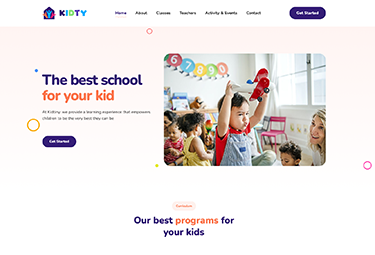The image has a white border at the top displaying the text "Kid TY." The accompanying text is quite small and blurry, rendering most of it unreadable; however, the visible sections include tabs labeled "Home," "About," "Teachers," and "Activity." Additionally, there is a dark blue button with the text "Get Started." 

The section below features a light pink background, with the slogan "The Best School" written in dark blue letters and "For Your Kid" in orange letters. To the left of this text is a blue dot, and below it to the left is an orange circle. Another dark blue button appears below this text.

To the right of the pink section is an image of a classroom filled with children. The classroom displays the number "67890" on the wall, has a window, and includes a smiling teacher who is looking at a child near the camera. The child, wearing a red shirt and overalls, has their arms raised in excitement.

At the bottom of the image, the text "Our Best" is written in dark blue letters, followed by "Program" in orange letters, and concluding with "For Your Kids" again in dark blue letters.